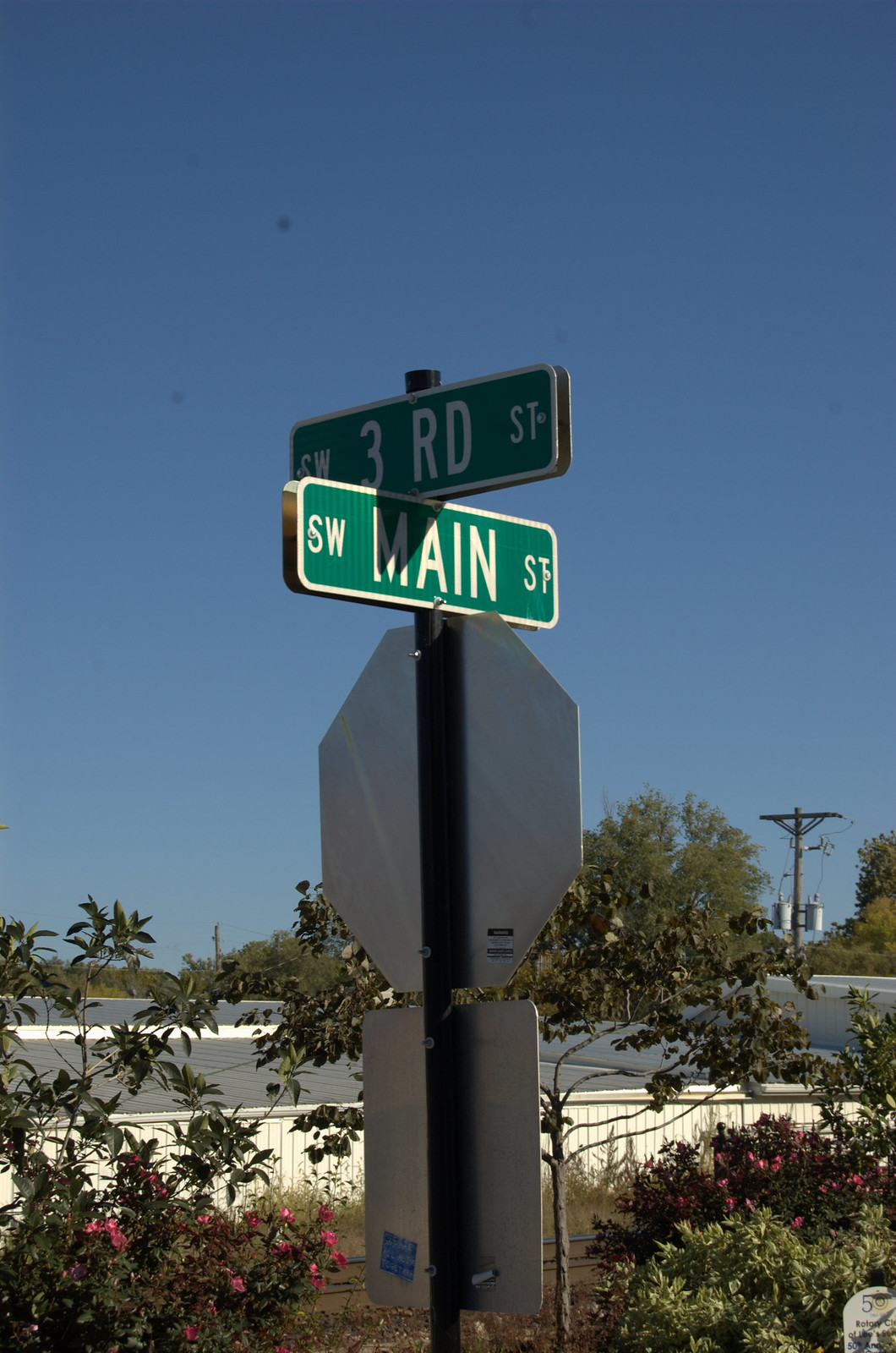The image features a street sign post at a crossroad, displaying two green street signs—Southwest 3rd Street at the top, running left to right, and Southwest Main Street below, extending forward and slightly to the right. Below the street signs, there is the back of a recognizable stop sign, followed by an unreadable rectangular sign that has a small blue sticker on it. Additionally, a black and white sticker is visible on the post. The backdrop includes lush vegetation, with a variety of trees and bushes, some adorned with pink flowers. Beyond the greenery, a white fence and a road border the scene, alongside a power pole with several transformers. The sky is a clear, vivid blue without any clouds, adding to the crispness of the image.